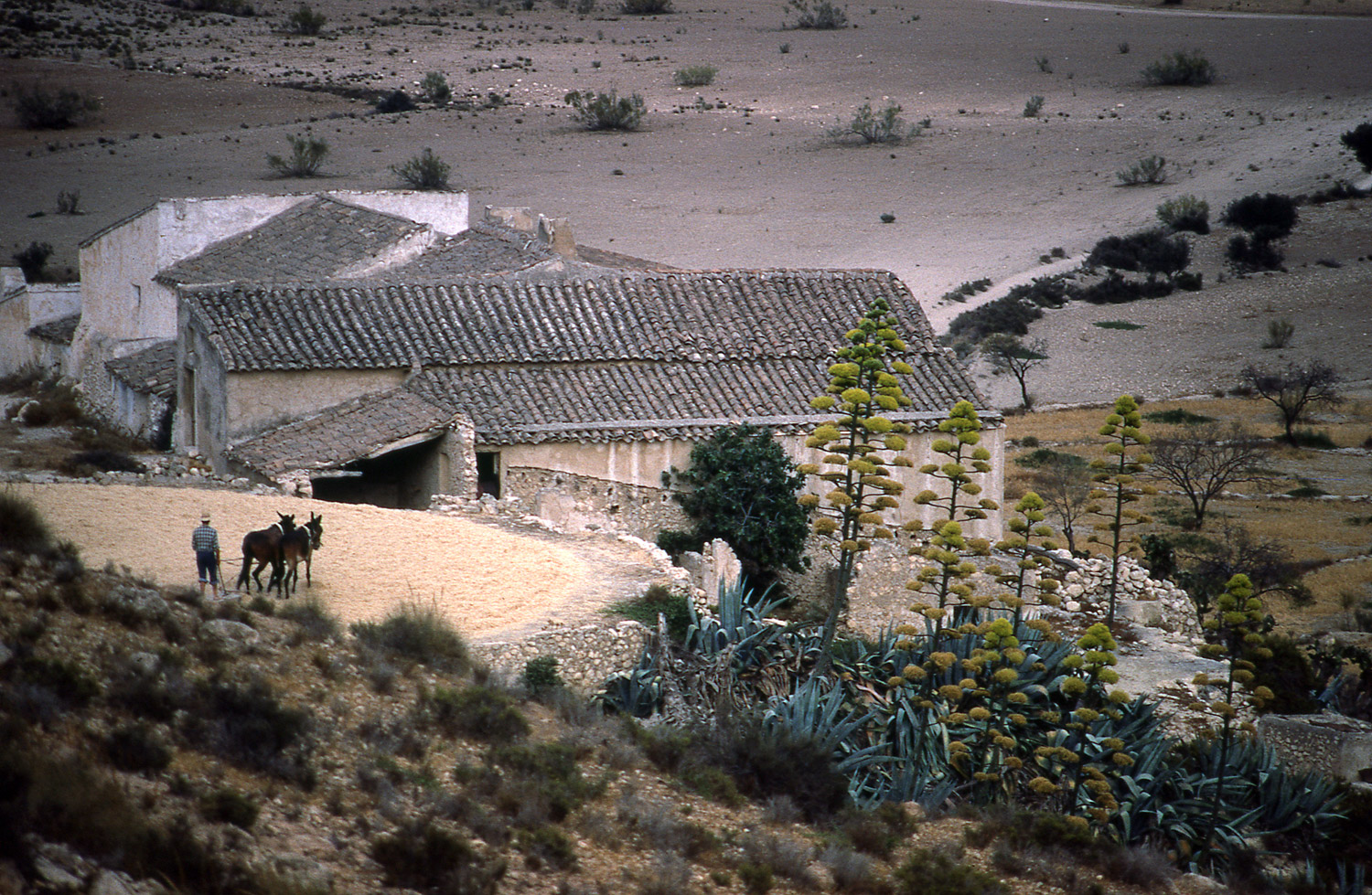In this image, a man in a blue shirt and blue jeans, adorned with a cowboy hat, stands in a broad, desert-like landscape, possibly in the Southwestern United States or Mexico. The man is walking behind two skinny animals, either donkeys or horses, which appear to be pulling something, suggesting he might be plowing the land. The animals have white or silver collars and are close together. The ground is flat and arid, with sparse vegetation including some cacti, brush-like plants, and tall plants with yellowish flowers. At the center of the image, there is a compound of buildings with clay or cement walls, some beige and others white, all topped with terracotta roofs. These structures, which resemble a ranch or a traditional house, look old and somewhat worn. The scene appears to be captured either near sunrise or sunset, giving it a dim, subdued feel. Although the sky is not visible, the overall ambience is one of quiet persistence in a rugged environment.